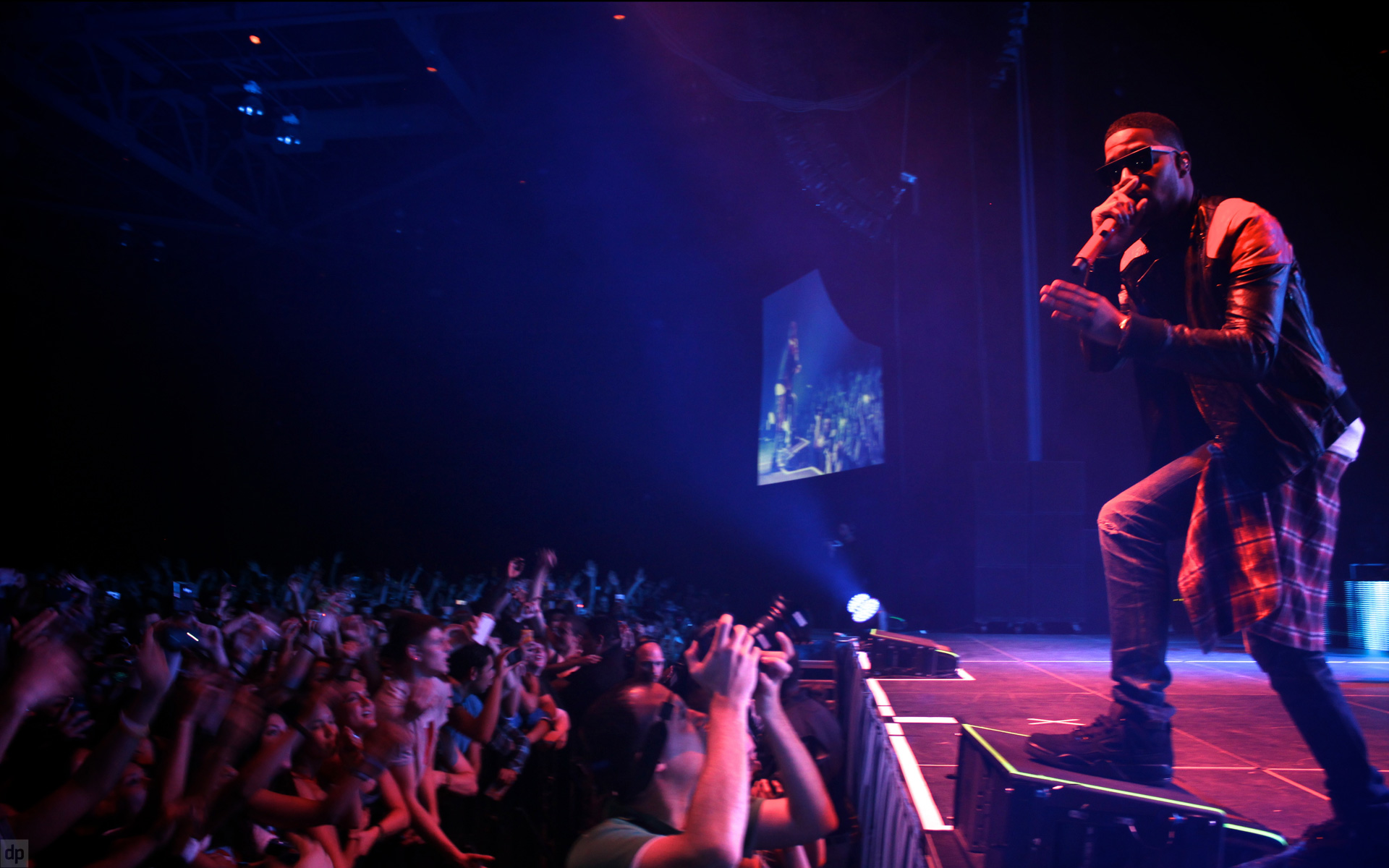The image showcases a vibrant live event or concert with an African-American male performer taking center stage. Dressed in a distinctive black leather jacket adorned with red and white on the shoulders, he also sports tight jeans and black shoes. A red and blue flannel shirt is tied around his waist, adding a nostalgic touch reminiscent of 90s fashion. His appearance is completed with square black sunglasses, and he holds a microphone in his right hand, suggesting he might be singing or beatboxing.

The stage is dramatically lit with red and blue lights, casting a dynamic atmosphere that contrasts against the pitch-black ceiling. The photograph captures the performer bathed in these lights, creating an intense and captivating visual. On the right side of the image and projected on a screen in the far background, the artist's performance is displayed for the audience members located further away, ensuring everyone has a clear view of the action.

The left side of the image features an enthusiastic crowd, packed and visibly excited, many with their hands raised in the air, cheering in response to the performance. The overall scene is one of energy and excitement, capturing the essence of a live concert experience.